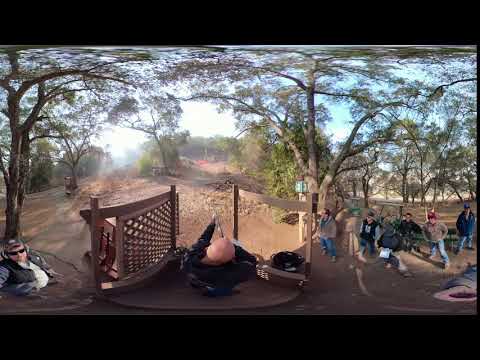The image captures a dynamic scene of a trap shooting event. A man is prominently positioned on a wooden platform, about 12 feet high and facing away from the camera, aiming his rifle towards targets at the base of a tall tree. The platform, complete with railing and latticework on the left, elevates him above the other participants. To the right of the platform stand seven men, all wearing ear protection, boots, and Levi pants. A single gentleman is also present on the left side of the platform, distinguishable in sunglasses, a black vest, and a light-colored undershirt, possibly observing or assisting. The ground below is a mix of brown and beige sand, indicative of a flat, open field. Tall trees surround the scene, contrasting with the sunny, clear sky peeking through their branches. The picture appears to be taken with a fisheye lens, offering a wide, slightly distorted panoramic view of the entire setup. Despite the bright sunlight, shade covers the area where most participants stand.